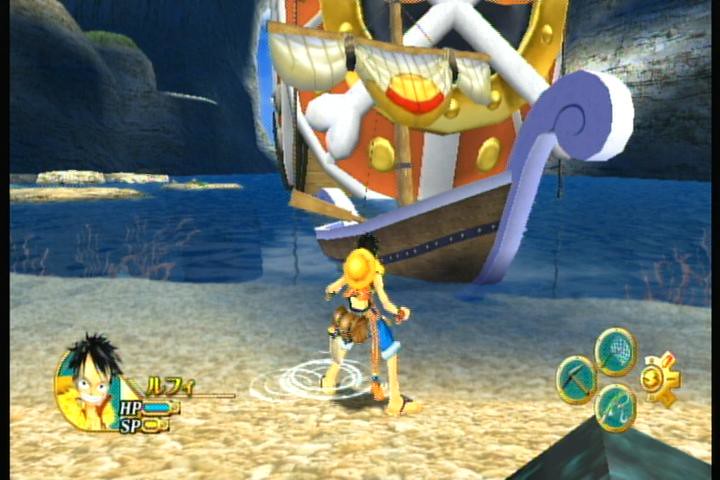The image depicts a screenshot from a video game set at a dark, eerie beach scene illuminated by a moon shining in a black, cloudy sky. The central character is a female cowgirl, identifiable by her large sun hat and substantial fanny pack. She stands with her arms outstretched on a sandy beach, gazing up at a colorful pirate ship docked nearby. The pirate ship, extravagantly decorated in hues of lavender, white, yellow, red, blue, orange, and gold, features a large barrel and traditional sails. A prominent logo in the lower left corner of the screen displays a clown face with wild black hair, marked with the character’s stats, "HP" with a blue bar and "SP" with a yellow bar. In the background, tall stone cliffs and smaller rock formations rise from the dark navy blue waters of a lagoon. Additional gameplay navigation buttons appear in the lower part of the screen, enhancing the immersive gaming experience.